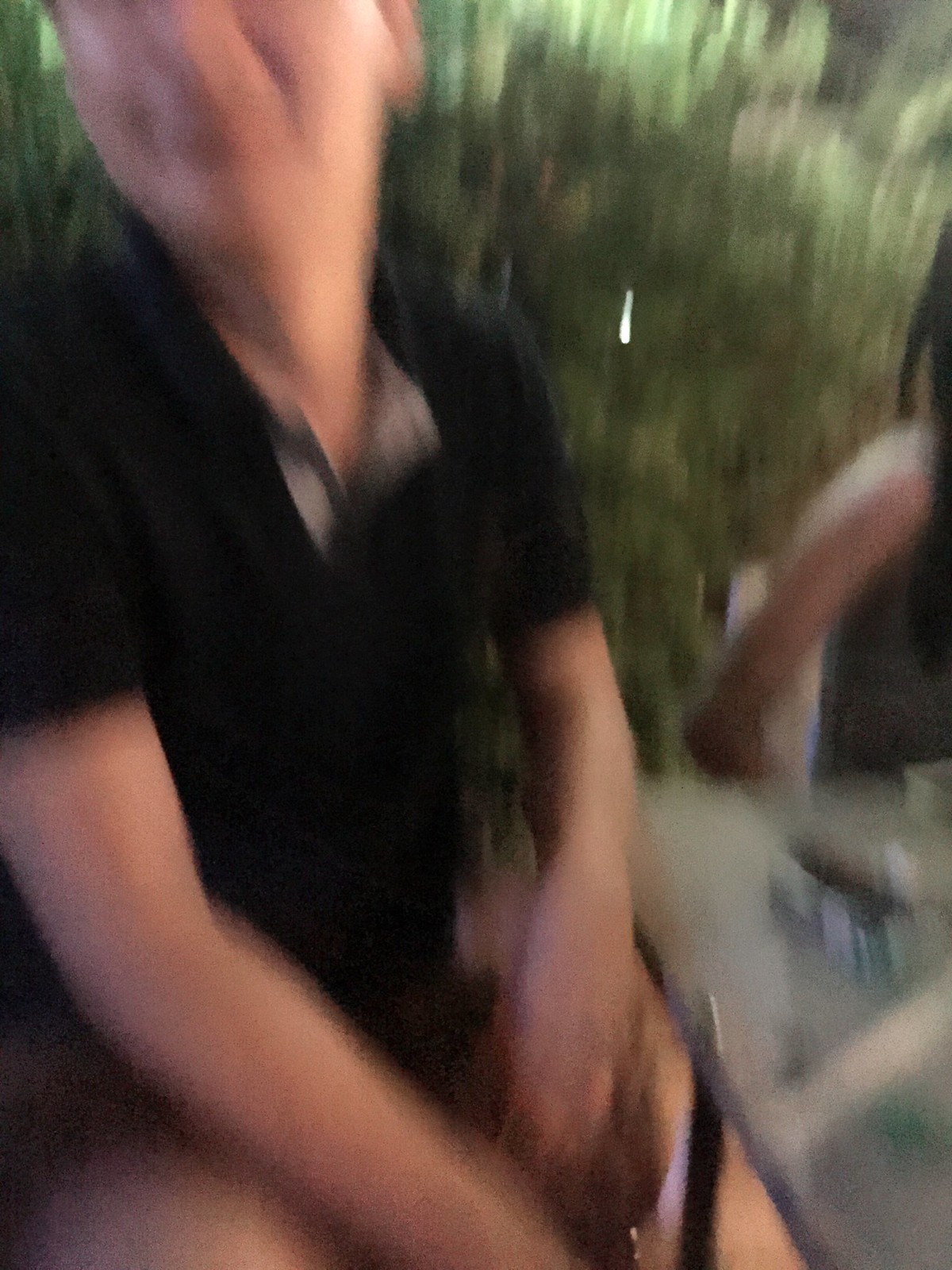The image is a photograph that is very blurry and out of focus, depicting a person in the foreground on the left side and a second person partially visible in the background on the right. The person in the foreground has fair skin and is seen from the tops of the ears and the bridge of the nose down to the thighs. This person is wearing a short-sleeved black shirt that is open at the collar, with some gray visible near the collar, possibly part of a buttoned detail. His upper thighs are bare, although it is not clear whether he is wearing shorts. He is seated next to a square or rectangular table, described by some as appearing gray and possibly having a glass cover.

To the very right side of the image, there is a partial view of another person with a dark complexion and dark hair styled in braids or locks. This person's visible features include their right arm and hair, which appears to be longer than shoulder length. They seem to be wearing a gray tank top, although one description mentioned a dark shirt. The background of the image suggests blurry vegetation, possibly bushes or trees. Overall, the photo captures a moment around a table set amidst a greenery backdrop, though much of the scene is indistinct due to the image's blurriness.